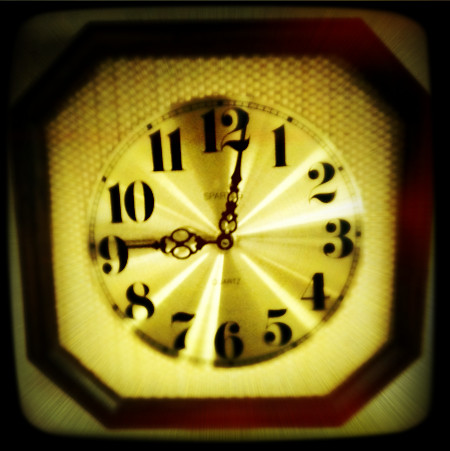This close-up color photograph captures a vintage-style clock, designed in an octagonal shape with clipped corners, giving it a total of eight edges. The clock face is a reflective, shiny gold with delicate black hands that are intricately designed with cut-out patterns. The time displayed is just after 9:01, marked by the black hour hand pointing to 9 and the black minute hand just past 12. Surrounding the golden clock face, a dark wood-like border provides a classic frame. The background features a tan woven fabric, adding to its antique appearance. Subtle text, partially visible at the top, and the word "quartz" at the bottom hint at its timekeeping mechanism. Glimmers of light reflect off the glossy surface, enhancing its delicate and elegant look.